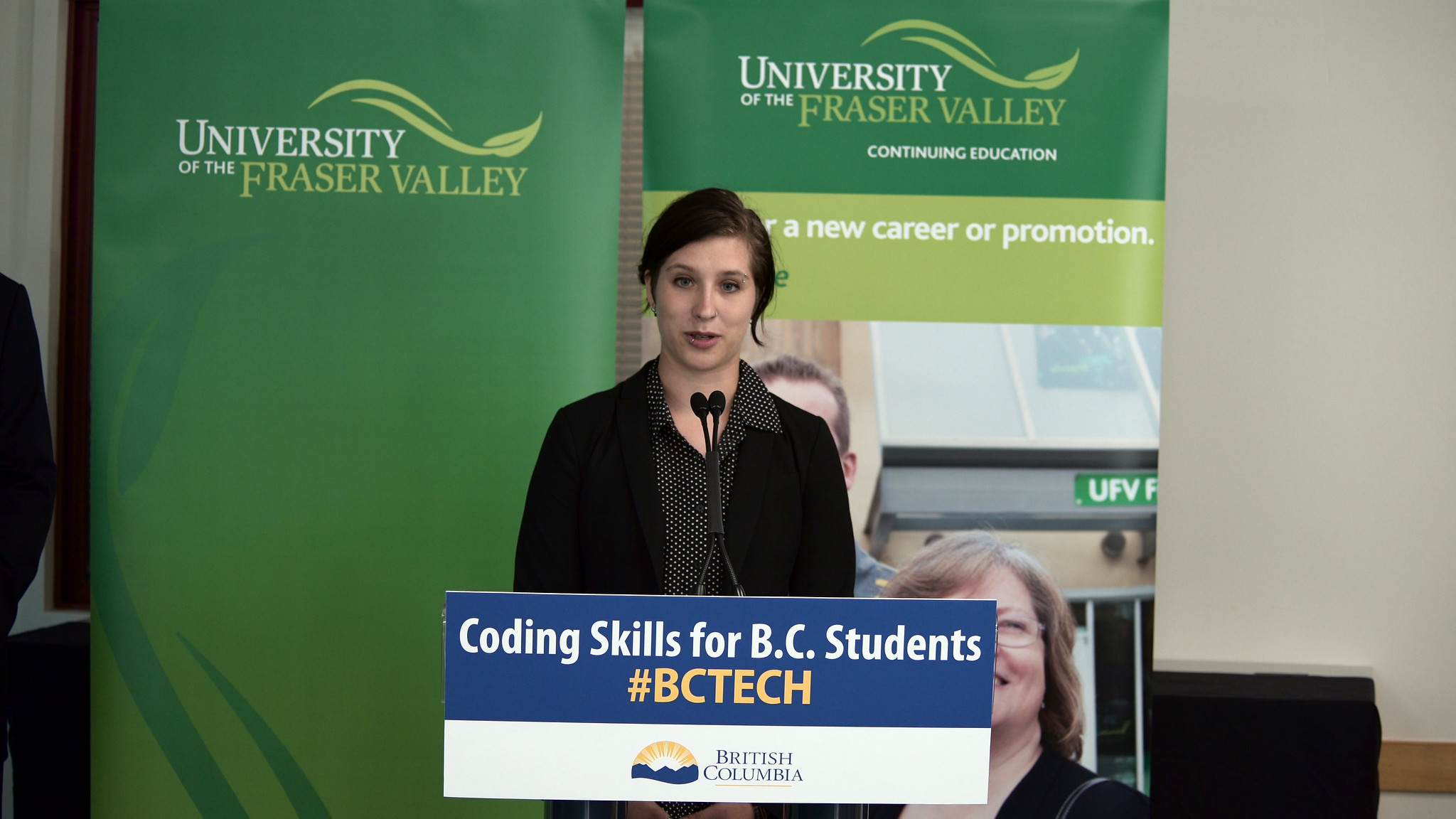The image features a young female presenter in her early 20s, standing at a centrally positioned podium with a microphone. Attached to the microphone is a sign that reads, in white text, "Coding Skills for BC Students" followed by the yellow hashtags "#BCTech." Beneath this text is the British Columbia logo, featuring a mountain silhouette with the sun on the horizon. Behind her, the backdrop consists of two green pull-up banners for the University of the Fraser Valley, one of which also mentions "University of the Fraser Valley Continuing Education" and displays an image of a female and male student. The setting is clearly indoors, with a simple white wallpaper background, and the event appears to be related to promoting new career opportunities at a university. The dominant color palette includes green, white, black, grey, blue, yellow, and tan.